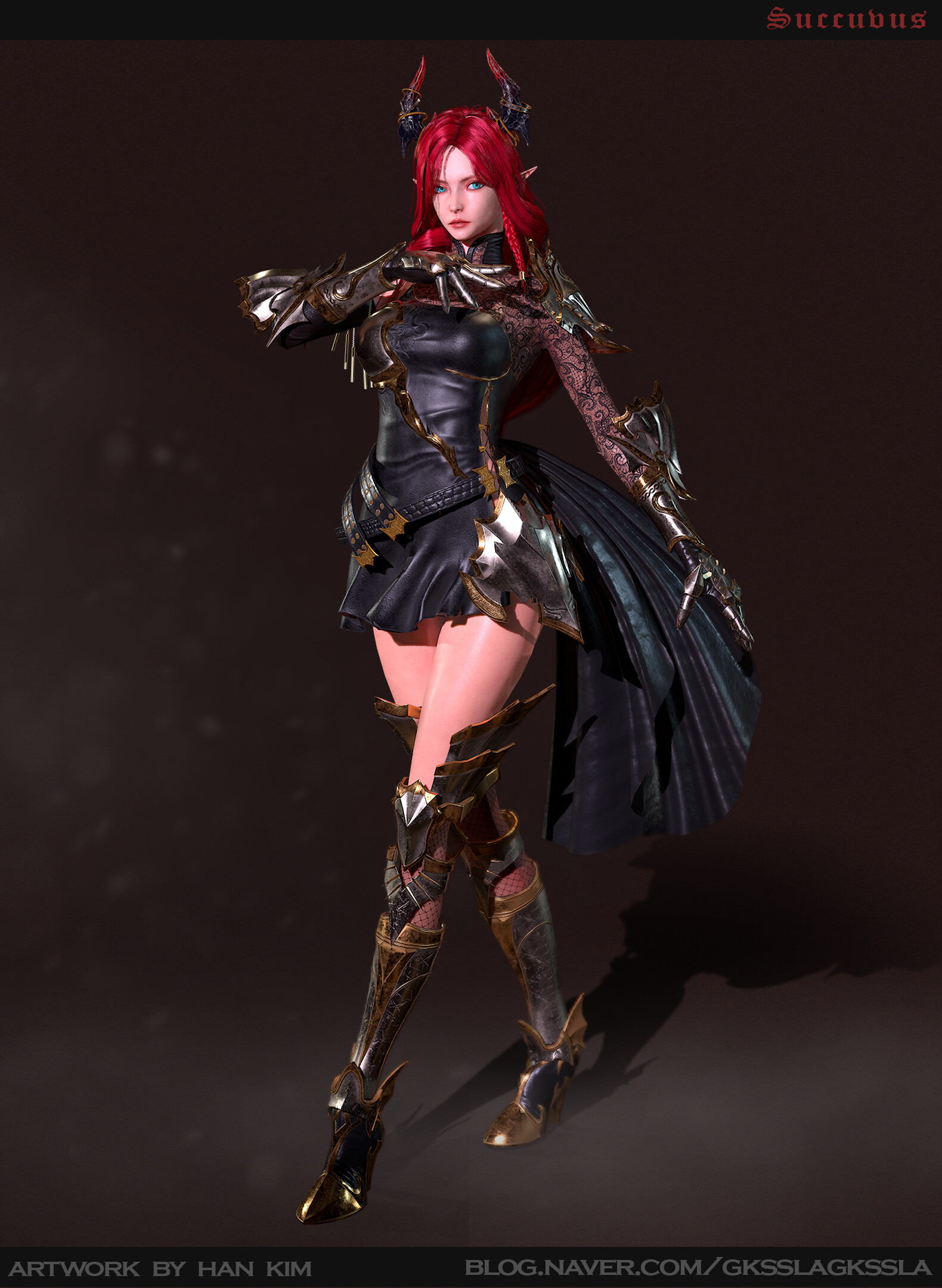The computer-generated image displays a striking female character with a fair complexion and vibrant red hair. She is dressed in an elaborate black leather outfit comprising a corset that extends from her chest to just about two inches down her thigh and knee-high armored boots with a metallic and brown hue. Her outfit is accentuated with metal gauntlet-styled gloves on her hands and forearms. She has two prominent black horns with red tips on her head, adding to her captivating appearance. The character is positioned with one arm raised towards the area above her breast and the other arm down, supporting a feather-like design at the back of her ensemble. 

The backdrop of the image is a consistent brown hue that seamlessly transitions from the floor to the background. Her shadow is visible against this backdrop, enhancing the depth of the image. In the upper right-hand corner, the word "Succubus" is clearly written in red font. The bottom of the artwork features the text, "Artwork by Han Kim, blog.naver.com/GKSSLAGKSSLA," acknowledging the artist and their blog. Different hues of black, deep red, maroon, light brown, off-white, tan, and flesh tones are notably present throughout the image, adding to the intricacy and allure of the character design.